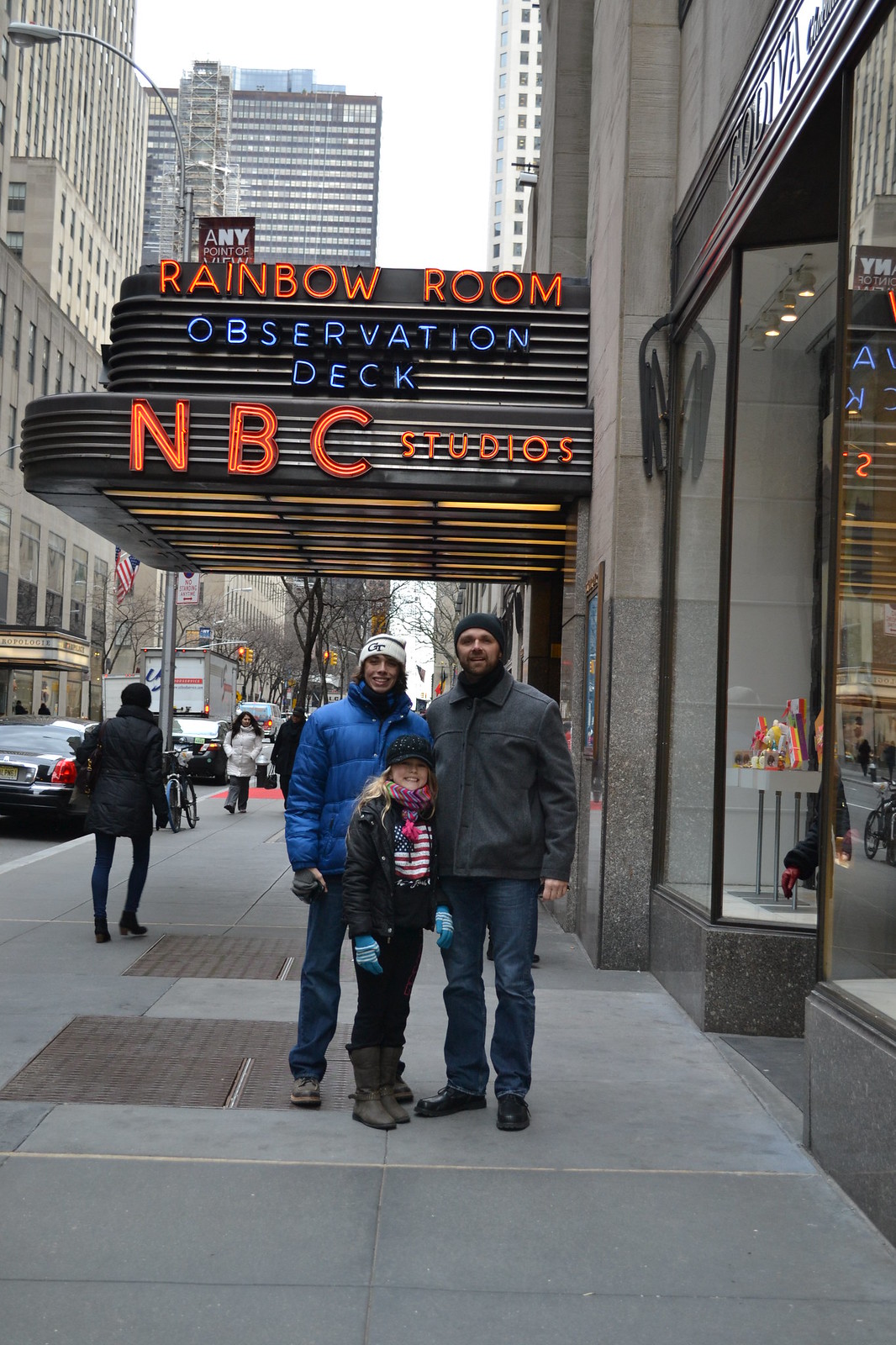In a bustling urban scene at Rockefeller Center in New York City, a family poses on the gray concrete sidewalk dotted with brown metal lids or grates, outside an NBC Studios glass storefront filled with various gift items on little shelves. Underneath the neon-lit awning displaying "Rainbow Room" in red, "Observation Deck" in blue, and "NBC Studios" in red, a woman stands on the left in a blue puffy jacket, blue jeans, gray shoes, and a beanie. Beside her, a man, presumably her husband, stands with their young child in the center, who is dressed in black pants, gray boots, and a black leather jacket. It's a cold season, likely fall or winter, as indicated by their winter coats and hats. The family smiles at the camera, surrounded by the iconic buildings of Rockefeller Center, while a few passersby and vehicles move along the cloudy, snow-free street. The edge of the photo reveals additional skyscrapers that frame this quintessential New York City moment.